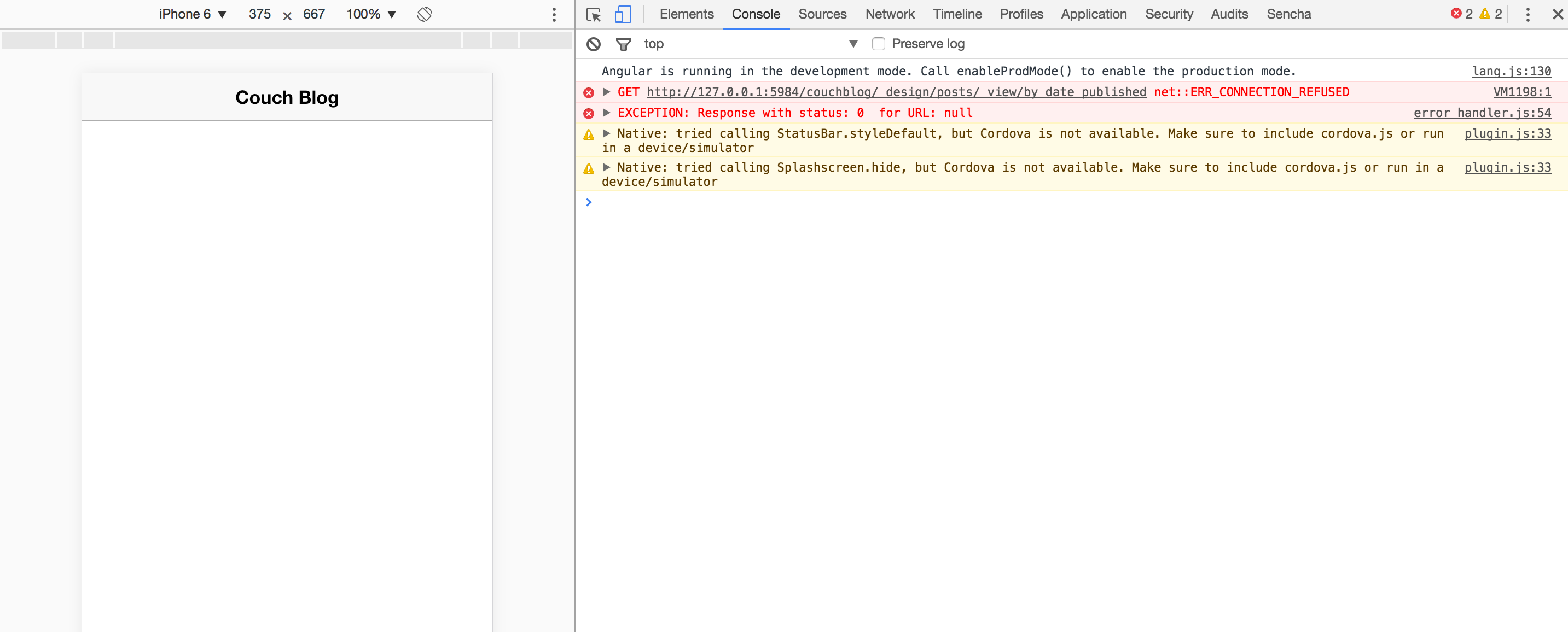The image is a detailed interface of what appears to be a digital platform or software screen.

- **Left-Hand Side:**
  - A small gray rectangle.
  - At the top, there are some words that are not legible.
  - Beneath the text is a darker gray line.
  - Below this line, there is a darker gray-outlined rectangle with the text "Couch Blog."
  - Underneath this, there's an empty white box.

- **Right-Hand Side:**
  - A collection of small symbols and words, which are difficult to make out due to their size.
  - A red dot with the number "2" next to it.
  - A yellow triangle with the number "2" next to it.
  - Three dots arranged vertically (one on top of the other).
  - An "X" icon.
  - A white rectangle featuring a series of symbols at the top, including a downward arrow and a gray-outlined square followed by some text.
  - Additional text beneath these symbols.
  
- **Middle Section:**
  - A pink box featuring a red circle with an icon inside it.
  - An arrow pointing to the right.
  - Text written in alternating colors: red, black, red, and black.

- **Lower Section:**
  - Another red dot with an arrow pointing to the right, followed by red text.
  - To the right of this, black text.

- **Bottom Portion:**
  - A yellow rectangle with a yellow triangle containing an icon and an arrow pointing to the right.
  - Black text interspersed with underlined black text.
  - Another yellow triangle with an icon, followed by an arrow pointing to the right and more black text.
  - Further black text on the right, also underlined.